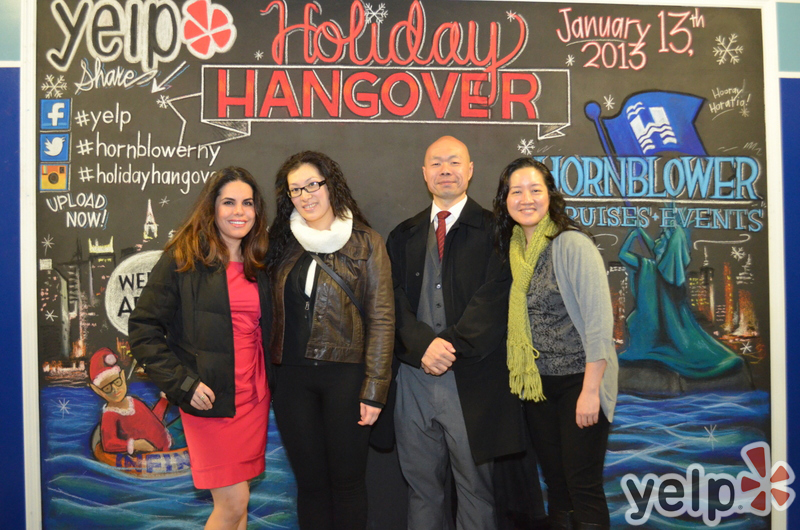The image showcases four individuals posing in front of a detailed and vibrant backdrop themed "Holiday Hangover." Central to the backdrop is a large black chalkboard-like display with a white frame, adorned with festive and corporate logos including Yelp, Facebook, Twitter, Instagram, and text such as hashtags for Yelp, Hornblower NY, and Holiday Hangover. Notable visuals include an elf floating in an inner tube on the left side and the Statue of Liberty holding a blue flag on the right, with the date January 13, 2013, and the words "Hornblower Cruises and Events" prominently displayed.

From left to right, the individuals include:
1. A woman with long brown hair, wearing a pink dress and a black puffer jacket.
2. Another woman, with curly black hair, outfitted in a brown leather jacket, black shirt, and black pants.
3. An Asian man, bald, dressed in a gray suit under a long black trench coat.
4. Finally, a woman with long brown hair, dressed in a gray top, gray sweater, black pants, and a long lime green scarf.

The setting captures an organized and celebratory moment, highlighting both the participants and the creative backdrop designed for the event.